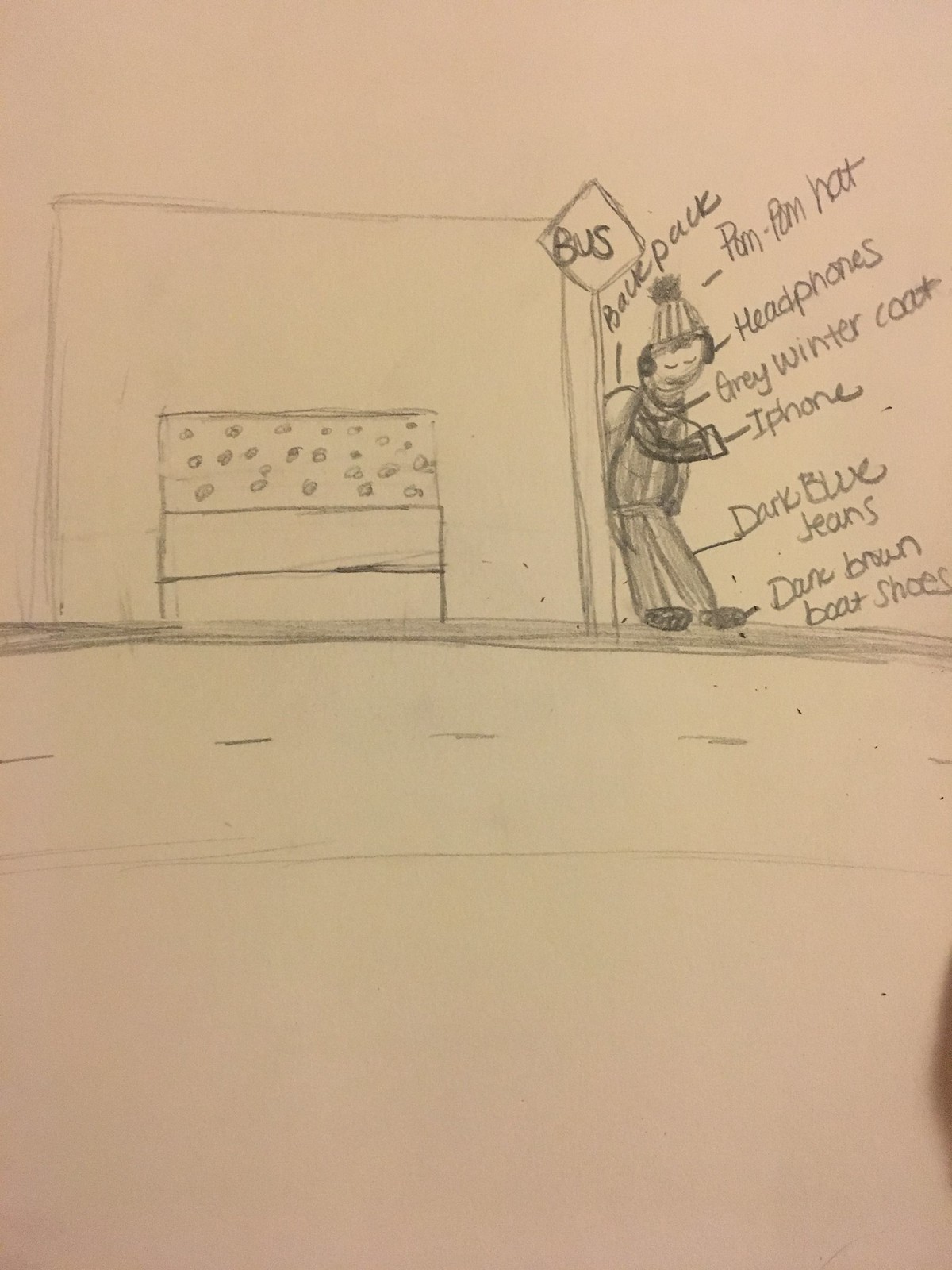The image is a child's crude sketch on light brown paper, approximately one and a half times taller than it is wide. It shows a simple scene composed of sketched lines and basic shapes. At the top of the image, a series of thick, horizontal lines run left to right, visually bisecting the paper. Below these lines, there is a dashed line followed by a solid line, representing a road with its divider.

On the left-hand side, a basic depiction of a bench is drawn using three stacked rectangles. Enclosing this bench, a larger rectangle signifies a building. Positioned at a bus stop sign, a figure is leaning against it. The sign is diamond-shaped with the word "BUS" inscribed on it, atop a long pole. 

The person standing near the bus stop is detailed with various labeled items, despite the overall simplicity. Wearing a beanie hat with vertical stripes and a pom-pom, headphones, a gray winter coat, and dark blue jeans, the figure's attire is meticulously described. They hold an object labeled as an iPhone in their hands. Around the figure are descriptive labels, clarifying each article of clothing and accessory.